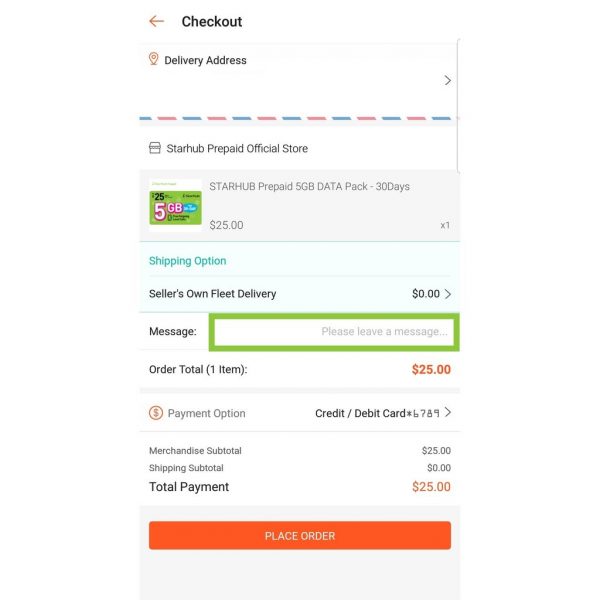This screenshot captures the checkout screen for an online order. At the top of the screen, there's a small orange arrow pointing left, next to the word "Checkout" written in black font. Directly below, a gray line separates the header from the main content. The first section displays "Delivery Address" with a right-pointing arrow on its far right. This is followed by a blue and red dashed line.

The next section features a white bar containing "Starhub Prepaid Official Store" in black font. Below this, a gray box provides details of the product: "Starhub Prepaid 5GB Data Pack, 30 Days." To the left of this text is a small logo resembling a gift card, while to the right, it states "$25" alongside "x1".

Following this, a light blue section indicates the shipping option. The text "Shipping Option" appears in blue, followed by "Sellers On Fleet Delivery, $0.00" in black, with a right-pointing arrow on the right. Lastly, there's a white background area labeled "Message." The input field here, outlined in green, contains placeholder text inviting the user to "Please leave a message."